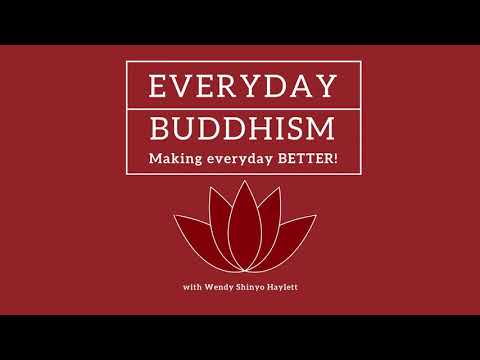The image features a predominantly burgundy background with black horizontal bars at the top and bottom. Centrally, there is a prominent red rectangle containing various elements. At the top of this rectangle, a thin white-lined box is divided by a horizontal line. In the upper half of this box, the word "EVERYDAY" is displayed in white capital letters, while the lower half contains the word "BUDDHISM," also in white capital letters.

Below the box, a tagline reads: "Making Every Day Better," with "Better" emphasized in all capital letters and an exclamation point. Beneath this tagline, there is an intricate red lotus flower design outlined in white, consisting of a central pointed petal flanked by pairs of petals extending outward on either side.

At the very bottom, in small white font, the text reads: "With Wendy Shinyo Haylett," attributing the image. The layout and colors—primarily black, red, and white—suggest a sophisticated and elegant design, reminiscent of a presentation slide or a promotional poster.